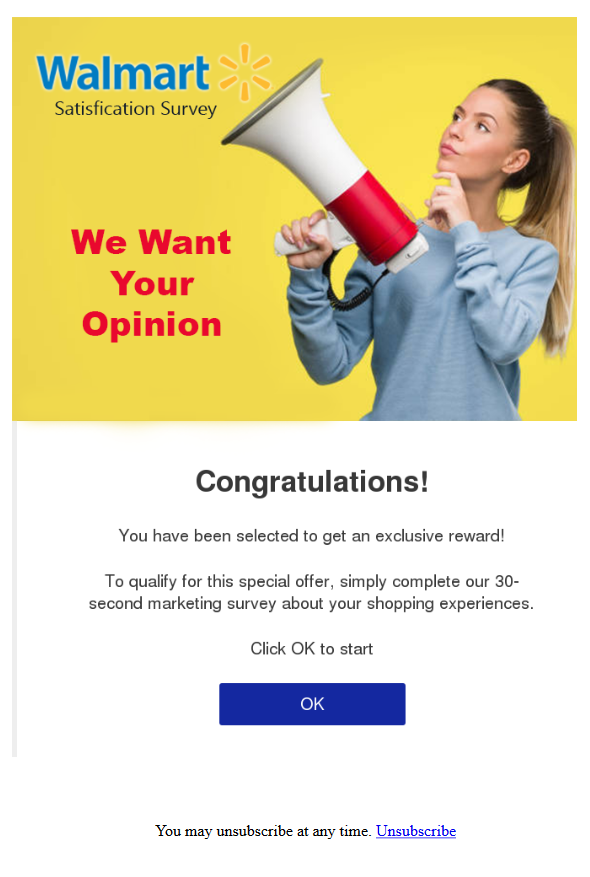This website section is designed to gather customer feedback through a satisfaction survey. The upper half features an orange square with the word "Wal-Mart" prominently displayed in blue letters, accompanied by the phrase "Satisfaction Survey" beneath it. Additionally, there is a small sunshine logo characteristic of Wal-Mart's branding. Below this header, in bold red letters, is the call-to-action message: "We want your opinion."

Within the orange square, there is an image of a woman. She is slightly tilting her head back, with one finger thoughtfully placed on her chin, holding an oversized red and white megaphone in her right hand, which also has a yellow handle. The woman, who sports a long ponytail and is dressed in a blue shirt, appears to be staring into the distance, reinforcing the thoughtful and engaging theme of the survey invite.

Beneath the image, the text reads: "Congratulations! You have been selected to receive an exclusive reward. To qualify for the offer, simply complete our 30-second marketing survey about your shopping experiences." Following this, there is a blue button labeled "OK" to initiate the survey. Below the button, there is a notification stating, "You may unsubscribe at any time," accompanied by a link to opt out of future communications.